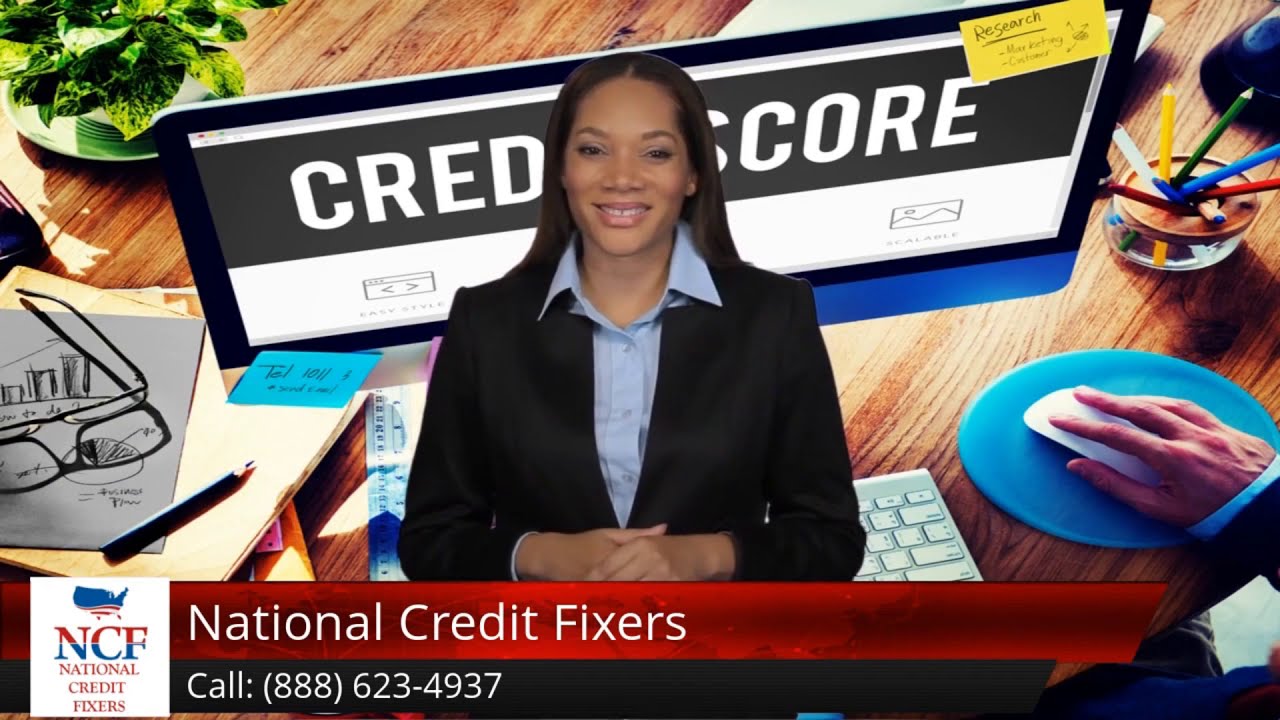The image is a screenshot from a commercial for National Credit Fixers, featuring a woman in a black suit jacket with a blue collar shirt underneath. She is an African-American woman with long black hair, clasping her hands together in front of her and smiling. Behind her is a typical office scene with a wooden table cluttered with various items including a pair of glasses, folders, colored pencils in a container, a pencil, sticky notes (one yellow with the words "credit score" in white font on a black background), a plant, and a computer setup with a keyboard and mouse, with a hand using the mouse. The background includes a black picture frame with white stripes and other office supplies. At the bottom of the image, there is a red banner with white text reading "National Credit Fixers" and underneath it in a white box, "Call 888-623-4937" in white font against a blue background. This is an advertisement for National Credit Fixers (NCF).